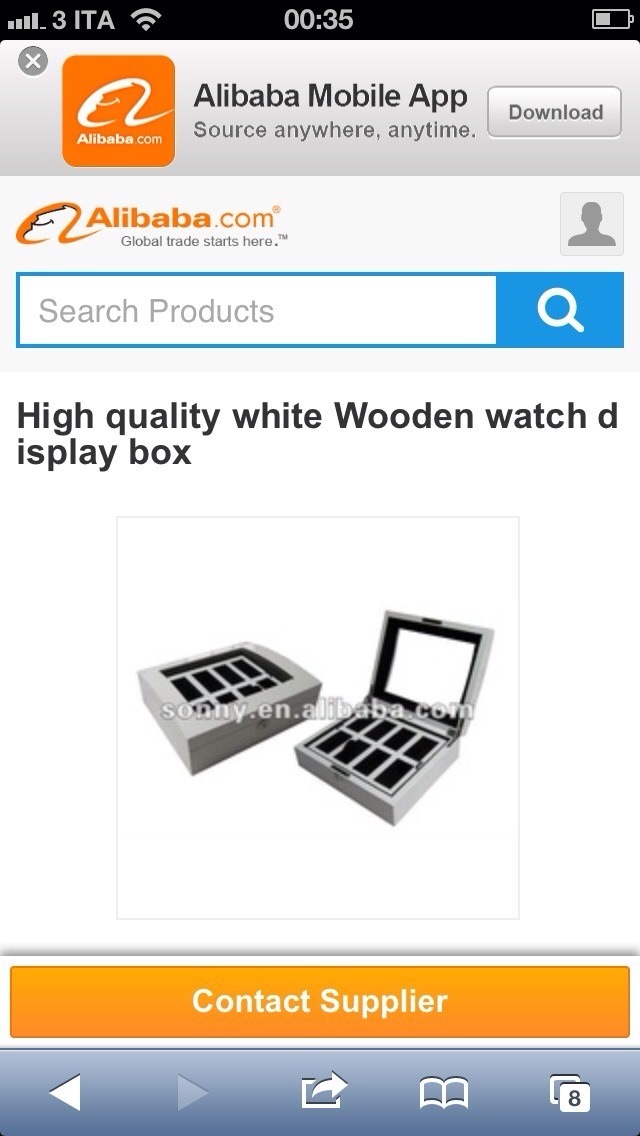The image appears to be a screenshot from a mobile phone and showcases the Alibaba mobile app interface. At the very top, there is a black border displaying cell service indicator "3ITA," a Wi-Fi signal icon, a time reading "00:35," and a half-charged battery symbol. Below this, the screen highlights the Alibaba mobile app slogan: "Source anywhere, anytime. Alibaba.com - Global trade starts here."

Further down, there's a blue search bar with the text "Search products," accompanied by a magnifying glass icon. In the main section of the screen, the product being advertised is a "High-quality white wooden watch display box," which is shown in an image. The box is white with a glass lid and can hold eight watches, visible through individual black slots when the lid is closed.

Beneath the product description, a prominent orange rectangular button labeled "Contact Supplier" is displayed in white text. At the bottom of the screen, a gray navigation bar features various symbols including a triangle, a forward button, and an open book icon, likely indicating additional pages or navigation options.